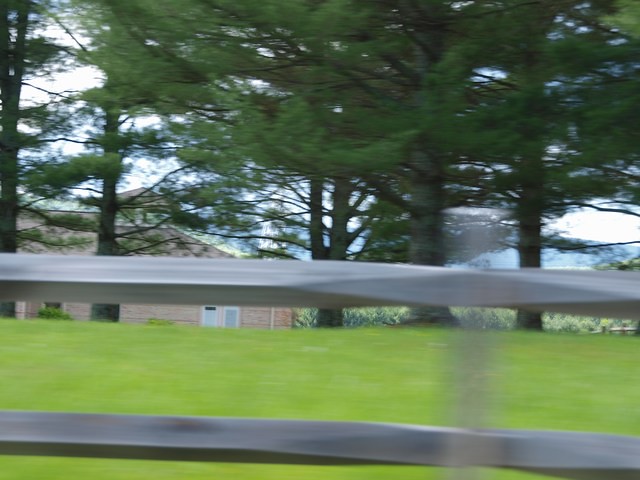The photograph captures a pastoral scene featuring a beige building in the distance, framed by lush, dark green trees with large trunks. In the immediate foreground, we stand beside a slightly blurry wooden fence, which has two horizontal posts that lead the eye into a field of rich greenery. The field extends towards the distant building and trees, under a bright sky. Far in the background, a faint outline suggests a possible small mountain or hill, adding to the scenic depth of the image.